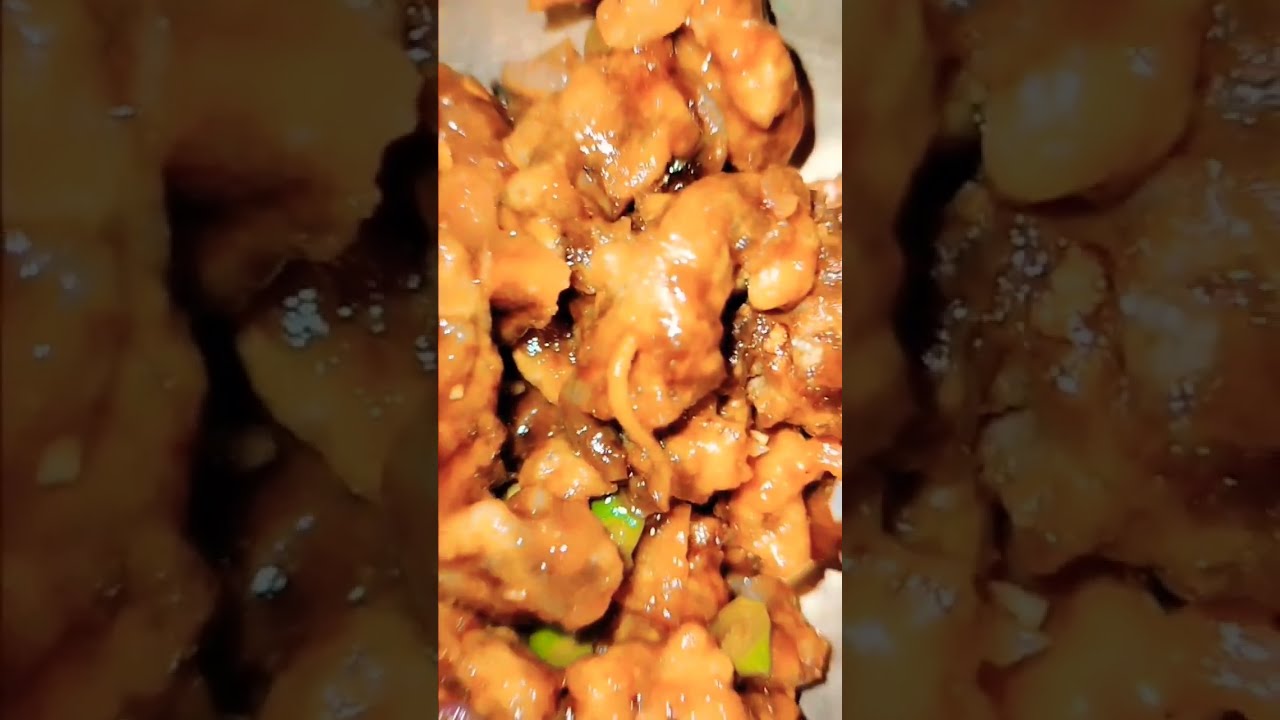This image features a close-up of what appears to be a delectable Chinese dish, possibly General Tso's chicken or sweet and sour chicken. The dish consists of bite-sized pieces of chicken coated in a glossy, brown glaze, giving it a mouthwatering appearance. Sprinkled throughout are green vegetables, likely green onions or green peppers, adding a splash of color and freshness. The food is presented on a white plate, which serves as a clean backdrop to highlight the vibrant elements of the dish. The overall image is divided into three horizontal sections of equal size. The left and right sections are darkened and appear to be zoomed-in versions of the central panel, albeit with an overlay of brown that makes them less distinct. These sections also seem to show the same pieces of chicken with small white specks that could be garlic, reinforcing the flavorful and savory appeal of the meal.